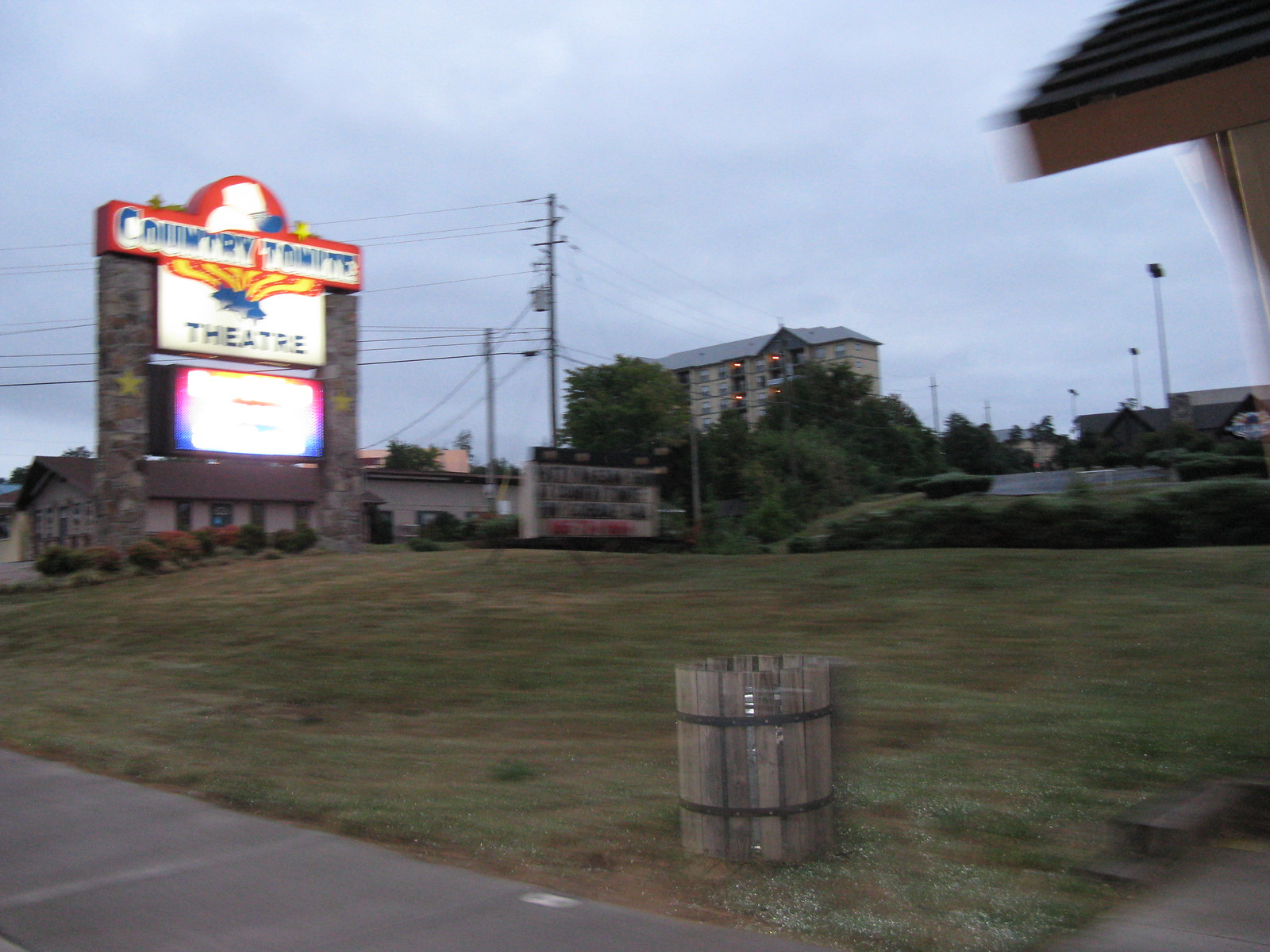In this rectangular landscape image taken at dusk, we see a scene from a sidewalk. Central to the image, there's a grass field with a slight slope, and prominently in the foreground, a wooden trash bin styled like a barrel with black metal rims. To the left of the grass, a tall, illuminated pylon sign for the "Country Tonite Theater" stands out. The top section of the sign is red with blue lettering spelling "Country Tonight" (stylized as T-O-N-I-T-E), the middle section is white with black letters spelling "Theater," and the bottom section, although blurry, has a white background with violet and blue rims. This sign is supported by two stone columns featuring yellow stars. In the background, slightly to the right, there’s a partly visible rectangular white monument sign with black plastic letters arranged in rows, though the text is unreadable. Behind these signs, a two-story inn with a brown rooftop is visible, as well as a taller hotel building. Electrical lines and poles are also seen in the distance, threading through the blue and white sky, adding to the intricate details of this outdoor scene.